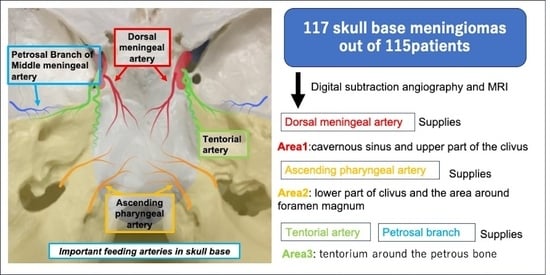This image is a detailed medical diagram depicting the interior of the skull, focusing on the various important feeding arteries at the skull base. On the left side, a photograph showcases several color-coded arteries, each accompanied by corresponding labels and arrows. The dorsal meningeal artery is highlighted in red, the tentorial artery in green, the petrosal branch of the middle meningeal artery in blue, and the ascending pharyngeal artery in yellow. The photograph features a white and mustard yellow material, with the white material positioned at the top and the yellow material below, containing several holes from which the arteries branch out.

On the right side of the image, a text description explains these arteries in further detail. At the top, a blue rectangle with rounded corners contains the text: "117 skull base meningiomas out of 115 patients, digital subtraction angiography and MRI." Beneath this, a black arrow points to a red-labeled "dorsal meningeal artery," denoted as supplying area 1, which includes the cavernous sinus and the upper part of the clivus. Following this, yellow text describes the "ascending pharyngeal artery" as supplying area 2, covering the lower part of the clivus and the area around the foramen magnum. Green text details the "tentorial artery," and blue text explains that the "petrosal branch of the middle meningeal artery" supplies area 3, tentorium around the petrous bone.

At the bottom of the photograph, a blue box emphasizes "important feeding arteries in the skull base," ensuring clear identification and educational value. The color-coded text on the right side matches the colors of the arteries in the left-side photograph, providing a coherent guide for understanding the anatomical pathways and regions supplied by these critical arteries.